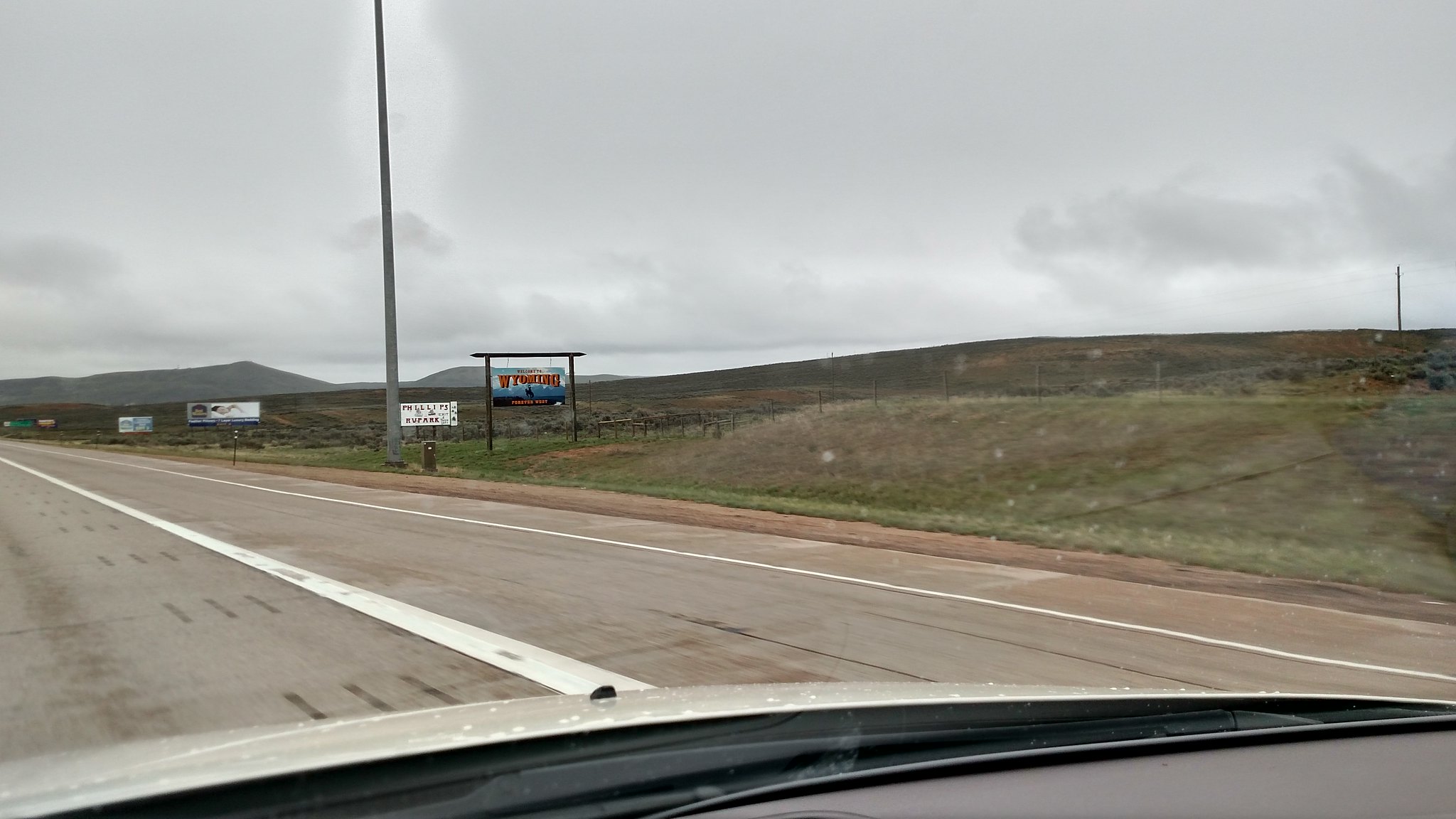The image is a landscape photograph taken from inside a vehicle, likely from the passenger seat, as indicated by the visible white hood, black dashboard, and a part of a windshield wiper on the bottom right-hand corner. The scene outside is an overcast, cloudy day, with a vast, desolate area featuring rolling hills and patches of grass and dirt along the highway. The road itself is gray, scuffed, and cracked, separated by white lane dividers. Off in the distance, towering grayish mountains loom under the cloudy sky. There's also a sign visible near the forefront, mounted on a brown post with a distinctive horizontal line on top, suggesting it might be a Wyoming sign against a blue background. The overall setting is sparsely populated, with hints of buildings emerging further along the route.